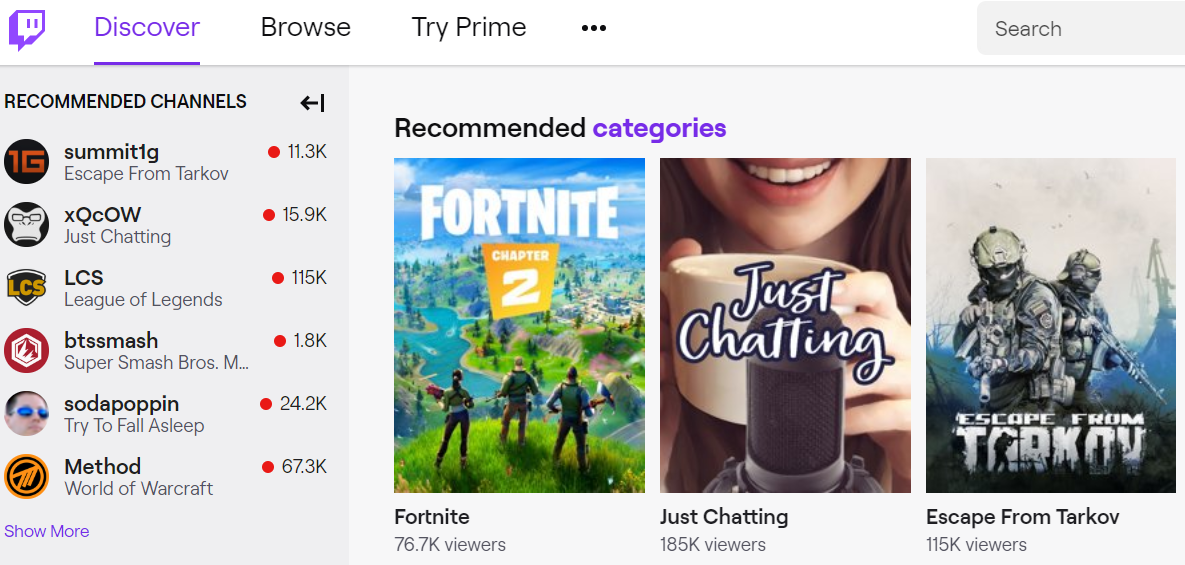This is a detailed descriptive caption for the given image:

---

The image is a horizontal screenshot of a Twitch menu interface. In the upper left corner, the familiar Twitch icon is prominently displayed. Below it, a white header bar stretches across the width of the screen, showcasing three main categories: “Discover,” “Browse,” and “Try Prime,” with "Discover" highlighted and underlined in purple. On the far right of this header, there is a grey search button located at the upper-right corner.

On the left-hand side of the screen, a vertical bar labeled “Recommended Channels” lists popular streamers, complete with their profile pictures and red dots indicating the number of posts, which number in the thousands. The highlighted streamers include Summit1G, XQCOW, LCS, BTS Smash, Sodapoppin, and Method.

The right-hand side of the screen features a section titled “Recommended Categories” with the word "Categories" written in purple text. Below it, three game categories are prominently displayed:
1. The first game listed is "Fortnite," accompanied by an image from Fortnite Chapter 2.
2. The second category, "Just Chatting," features an image of a woman holding a coffee cup in front of a microphone.
3. The final category, "Escape from Tarkov," is represented with an image of military men set against a grey, blue, and white illustrated background.

The image captures the clean and organized layout of Twitch's user interface, highlighting popular streamers and trending game categories.